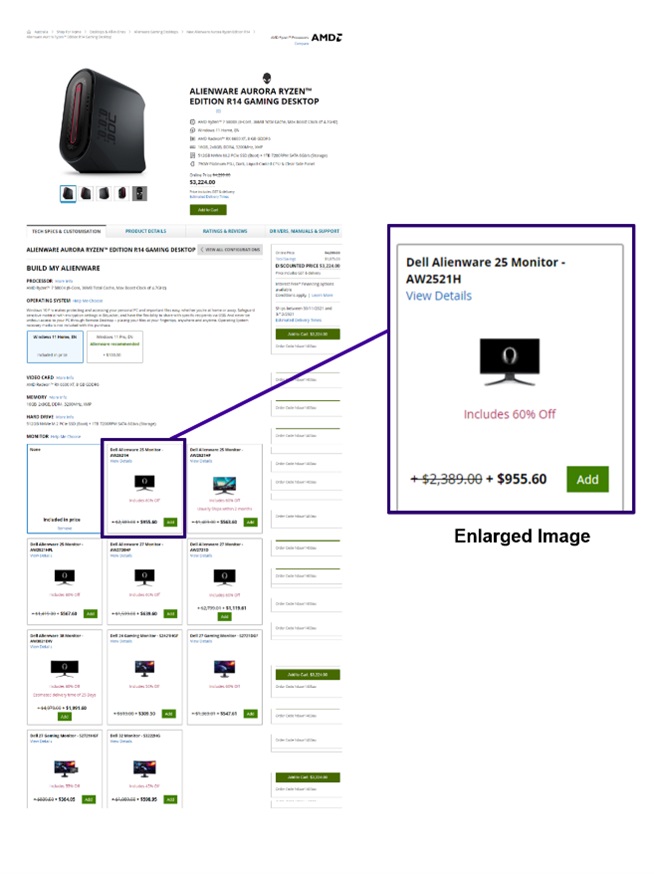This image showcases the Alienware Aurora R14 Gaming Desktop - Rising Edition, prominently highlighted by Alienware. Accompanying it is the Alienware 25 Monitor (Model: AW2521H), currently detailed with an impressive discount of 60%. Both devices are displayed together, presenting a harmonious gaming setup.

At the top right corner of the image, the AMD logo is clearly visible, indicating that the system is powered by AMD technology. Various customization options and specifications for the purchase system are summarized, including selectable colors: White, Black, Green, and Blue. However, the final price is not listed in this preview. The image is enhanced to provide a closer look, ensuring all details are clearly presented for potential buyers.